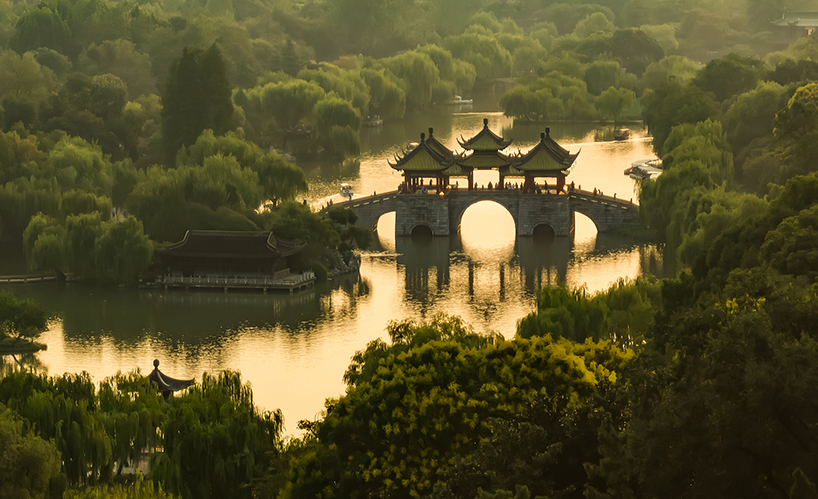A horizontal rectangular color photograph captures a serene and picturesque scene in China. The image features a stone pedestrian bridge adorned with three pagoda-like structures along its span, stretching over a tranquil yellow-tinted river that reflects the sunlight. The water is mostly still with just a few gentle ripples, creating a sparkling effect. Lush, vibrant green trees and yellow flowers surround the river, adding a burst of color and life to the setting. To the left of the bridge, a building, possibly a pier with a white fence, stands partially over the water. The majority of the scene is framed by dense forest, enhancing the peaceful ambiance of this natural and tranquil location.